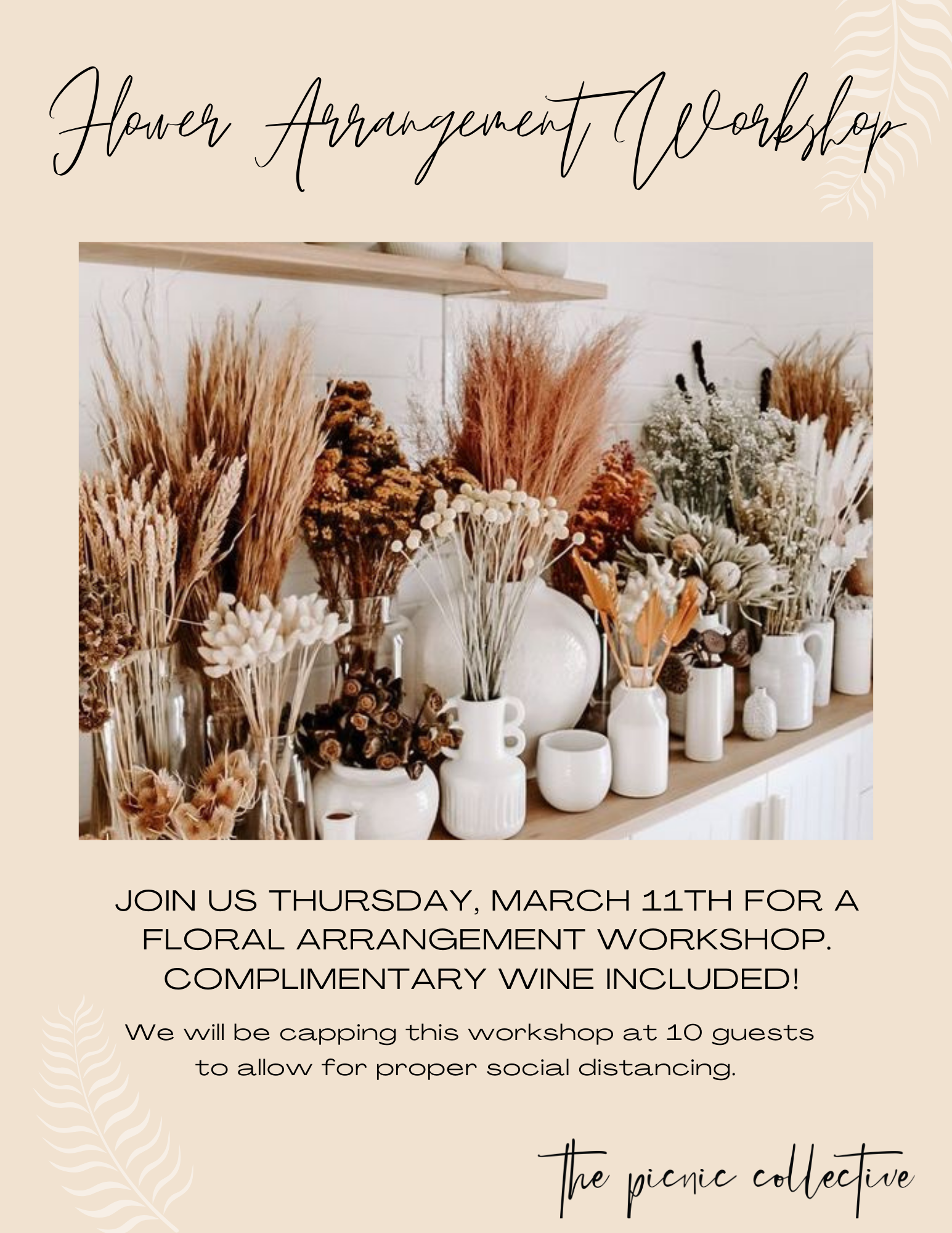Advertisement for a Flower Arrangement Workshop

This vibrant advertisement, set against a pale, pastel pink background, features elegant cursive text at the top that reads "Flower Arrangement Workshop." Below the ornate script, a central rectangular image showcases an artful display on a two-shelf wooden bench. The front shelf is adorned with white pottery vases of various shapes and sizes, each holding an assortment of dried flowers, grasses, and plants in shades of white, tan, and gray. The second shelf is filled with taller, more rustic dried grasses and reed stems in hues of brown and rust. Below the image, text in black letters invites viewers to join the workshop on Thursday, March 11th, with complimentary wine included. The workshop is limited to 10 guests to ensure proper social distancing. At the bottom of the poster, the event is signed off in cursive by The Picnic Collective.